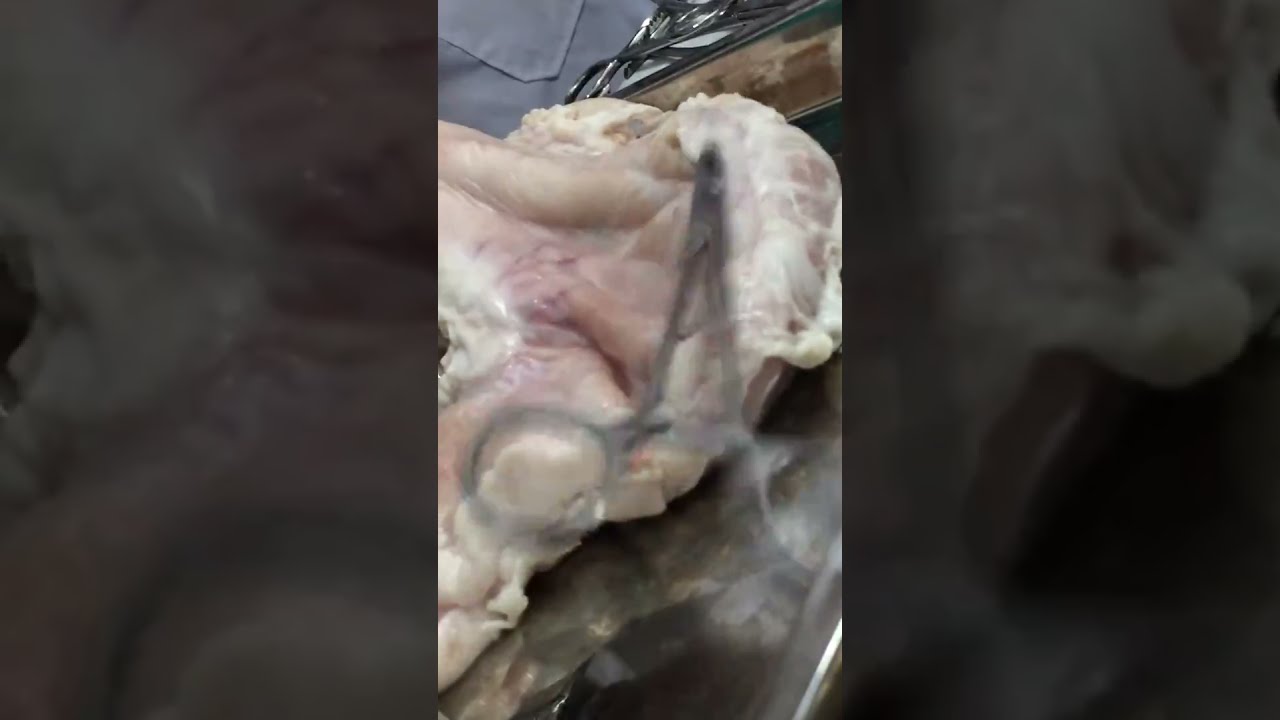This detailed photograph captures a medical scene where a pair of latex-gloved hands are meticulously performing a procedure. The primary hand in the foreground holds a pair of fine metal scissors, while the other hand, also gloved, deftly manipulates a black thread, sewing into a pale, whitish organ-like object. This object, possibly flesh or fat, has pinkish hues and cream-colored edges, giving it a lifelike quality. The thin, black stitches are clearly visible, meticulously stitching the organ on top of a metallic tray situated on a white table. Additional silver scissors rest on the organ, hinting at the intensity and precision of the task at hand. In the background, other medical personnel dressed in blue uniforms are faintly visible, though their focus remains on the central procedure. The image conveys the seriousness and concentration inherent in medical surgeries or dissections, with a stark black backdrop framing the scene.